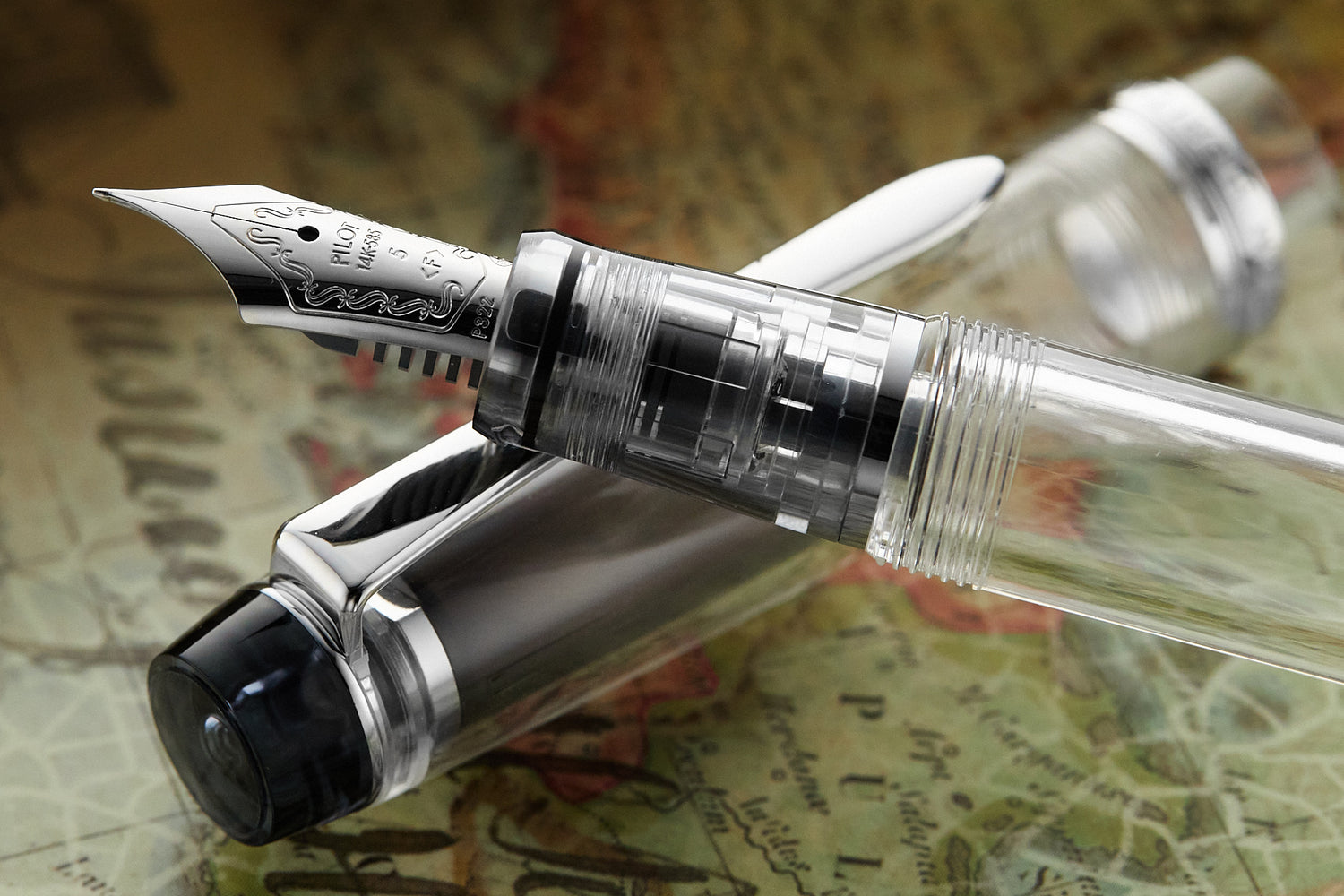This is a highly detailed, photorealistic macro shot of an elegant clear fountain pen, prominently showcasing its shiny silver triangular nib with intricate embossed filigree. The nib, inscribed with "Pilot 14K-505" and "5 (F)" along with "P822" in the corner, points towards the left side of the image. The pen, crafted with a clear plastic casing, extends from the right side of the frame and rests atop its cap, which features black and silver accents and a silver clip. Both the pen and the cap lay angled against each other on a map adorned with subtle colors of green, pink, and yellow, with terrain lines and cursive words that are too blurred to read. The image, likely intended for an advertisement, is artistically lit from the side to highlight the pen’s fine details and the vibrant map underneath, creating a visually striking and sophisticated composition.